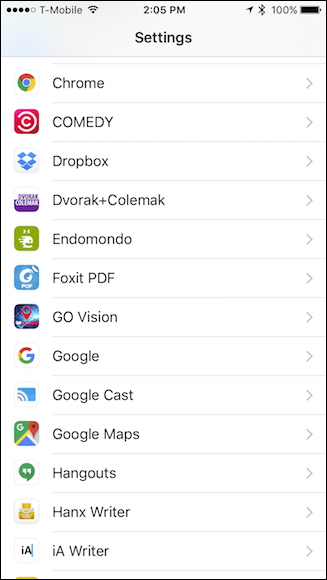The image appears to be a screenshot from a cell phone. At the top left corner, there are four out of five dots filled in black, indicating the signal strength. To the right of this, the word "T-Mobile" is displayed. The time is shown as 2:05 PM, and the battery life is at 100%. 

Below this, in black text, is the word "Settings" followed by several subcategories of apps and features. The first listed is "Chrome" for the Google Chrome browser, identified by its circular logo with red, yellow, and green segments. Next is "Comedy," represented by a red circle with the letter "C" inside.

Following this are the listings for "Dropbox," "Dvorak," and "Colmac," without specific icons described. The app "Endomondo" is marked by a green square. Below it, "Foxit PDF" is denoted by a blue square. Then there are listings for "Go Vision," "Google," "Google Cast," and "Google Maps," without specific icons mentioned.

"Hangouts" is next, featuring a green speech bubble with two white lines inside. Beside "Hanx Writer," stylized as "H-A-N-X-W-R-I-T-E-R," there appears to be the image of a printer. Finally, "IA Writer" is listed with an icon showing a lowercase 'i' next to an uppercase 'A'.